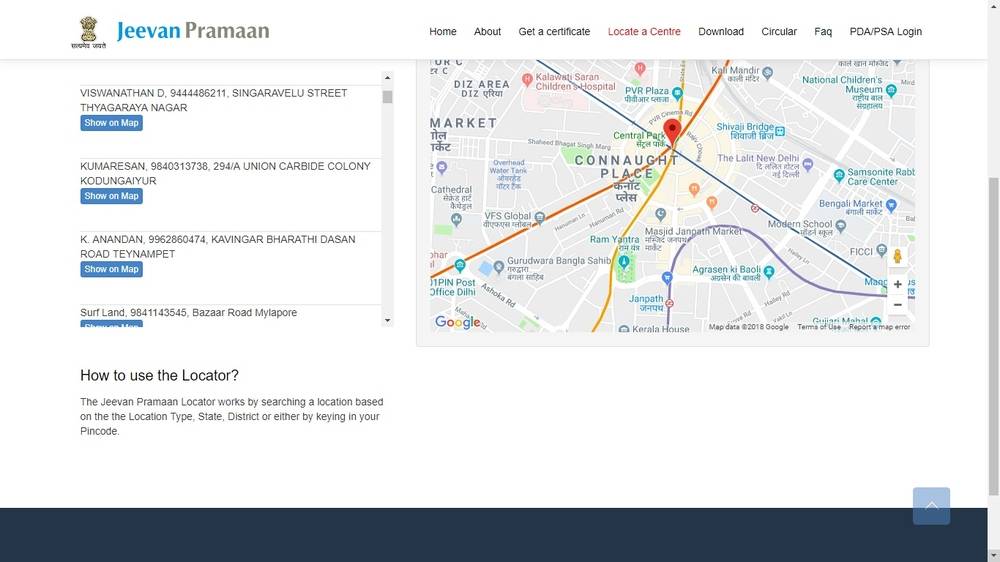This image is a screenshot from the Jeevan Praman website. In the upper left-hand corner, the name "Jeevan Praman" is prominently displayed alongside an icon that resembles a crown. 

Below the header, a list of names written in a different language can be seen on the left side of the screen. Each name is accompanied by a blue box that contains the option to "Show on Map." 

On the right side of the screen, a gray search bar allows users to scroll through selections that have been generated. This section explains how to use the locator, noting that the Jeevan Praman locator operates by searching for locations based on criteria such as type, state, district, or by inputting a pin code.

Above this interface, a navigation bar features various options such as "Home," "About," "Get a Certificate," "Locate a Center" (highlighted in red), "Download a Circular," "FAQ," "PGA," and "PSA Login." 

On the right side of the page is an interactive map, displaying key locations with a pin placed at a strategic point where main roads and interstates intersect, underscoring the site's accessibility.